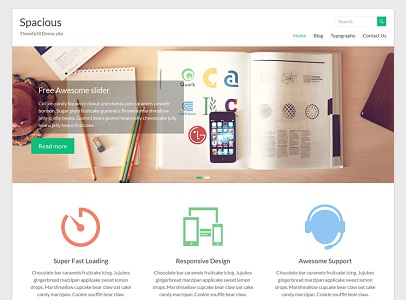This is a detailed description of a web page design.

The web page features a gray border surrounding all sides except the bottom. In the top left corner, the word "Spacious" is prominently displayed, followed by some blurred text below it, hinting at the phrase "demo site." In the top right corner, there is a search bar. Below the search bar, the navigation menu includes "Home," which is highlighted, followed by "Blog," "Typography," and "Contact Us."

The main section of the page showcases a full-width photo taken from an aerial view. The photo features a notepad with writing and a few pencils, an open book, and a cell phone displaying various app icons. Overlaying this image is text reading "Free Awesome Slider," accompanied by several lines of out-of-focus text, and a green rectangle button labeled "Read More."

Beneath the main image, there are three distinct icons. The left icon shows a red stopwatch or clock with the label "Super Fast Loading" and some blurred text underneath. The middle icon, displayed in green and white, depicts a larger cell phone, a computer monitor, and a smaller cell phone, representing a "Responsive Design" with some additional blurred text below it. The rightmost icon features a person’s head wearing earphones, labeled "Awesome Support," also followed by some out-of-focus text.